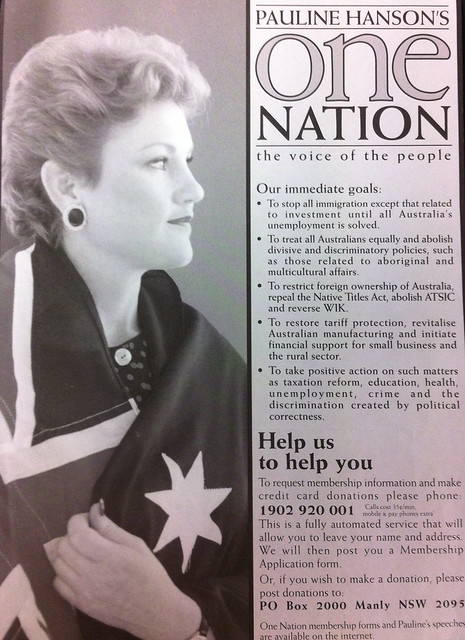This black and white political advertisement features a woman, identified as Pauline Hanson, on the left side, draped in what appears to be the British flag. She has short, thick hair and is wearing large, noticeable earrings. The image is part of a campaign poster for Pauline Hanson's "One Nation," with the slogan "The Voice of the People" prominently displayed at the top. The right side of the poster lists several political goals, including stopping all immigration except for investment-related purposes until Australia's unemployment is resolved and promoting equality among all Australians by abolishing divisive policies affecting Aboriginals and multicultural affairs. The bottom section of the poster invites viewers to request membership information and make credit card donations, providing a phone number, address, and further contact details for this purpose.